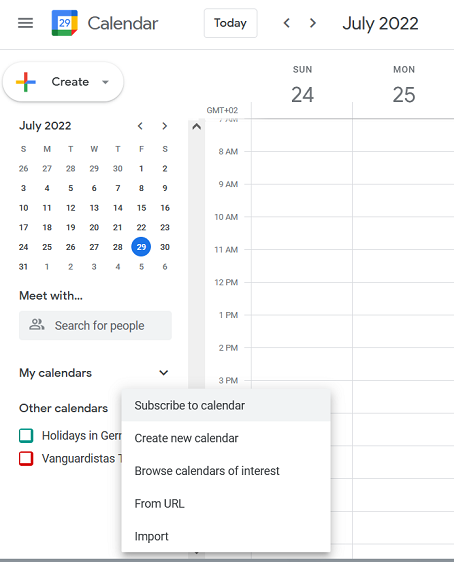This image depicts a detailed interface of the Google Calendar app. Dominating the top portion of the screen, the header features the Google Calendar identification prominently. On the top left, the word "Calendar" is visible, flanked by the familiar Google logo—encased in a square with the number "29" inside. Beside the Google logo on its left, a hamburger menu icon is situated, providing additional navigation options.

Located at the top center is the word "Today," accompanied by navigational arrows on either side, allowing users to skip forward or backward between dates. The top right corner showcases the current month and year, specified as "July 2022."

The middle left section of the image features the calendar layout for July 2022. The current day, the 29th, is distinctly highlighted within a blue circle, with the date marked in white text. Above the calendar, a "Create" button is clearly displayed. This button is marked with a multicolored plus symbol—red on the top, yellow on the left, green on the bottom, and blue on the right—indicating the functionality to add new events.

Below the calendar, a search box labeled "Meet with" invites users to "Search for people," enabling easy scheduling of meetings. Toward the very bottom of the interface, two more categories are visibly detailed: "My calendars" and "Other calendars." Under "Other calendars," options such as "Holidays in general" and "Vanguard sisters" are listed, providing organizational and additional event options for the user.